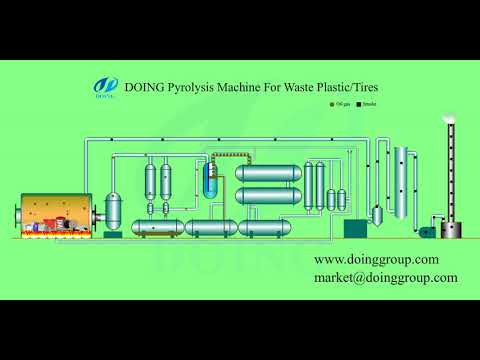This landscape-oriented image features a detailed color illustration set against a bright lime green background, bordered on the top and bottom by wide horizontal black bars. At the top center, in black capital letters, is the headline "DOING PYROLYSIS MACHINE FOR WASTE PLASTIC/TIRES," accompanied by a logo to the left, which has a stylized 'S' shape in dark blue and light blue. The central illustration depicts a pyrolysis process with intricate machinery, including various cylindrical metal gray tanks and interconnected pipes. On the left side, there is a gold-colored elongated container emitting bubbles, while on the right side, a vertical tower with a flame at its apex signifies the endpoint of the process. At the bottom right, the contact information is clearly displayed in black text: "www.doinggroup.com" with the email "market@doinggroup.com" directly underneath. The overall style of the image resembles a flowchart, visually detailing the pyrolysis machine's operation.